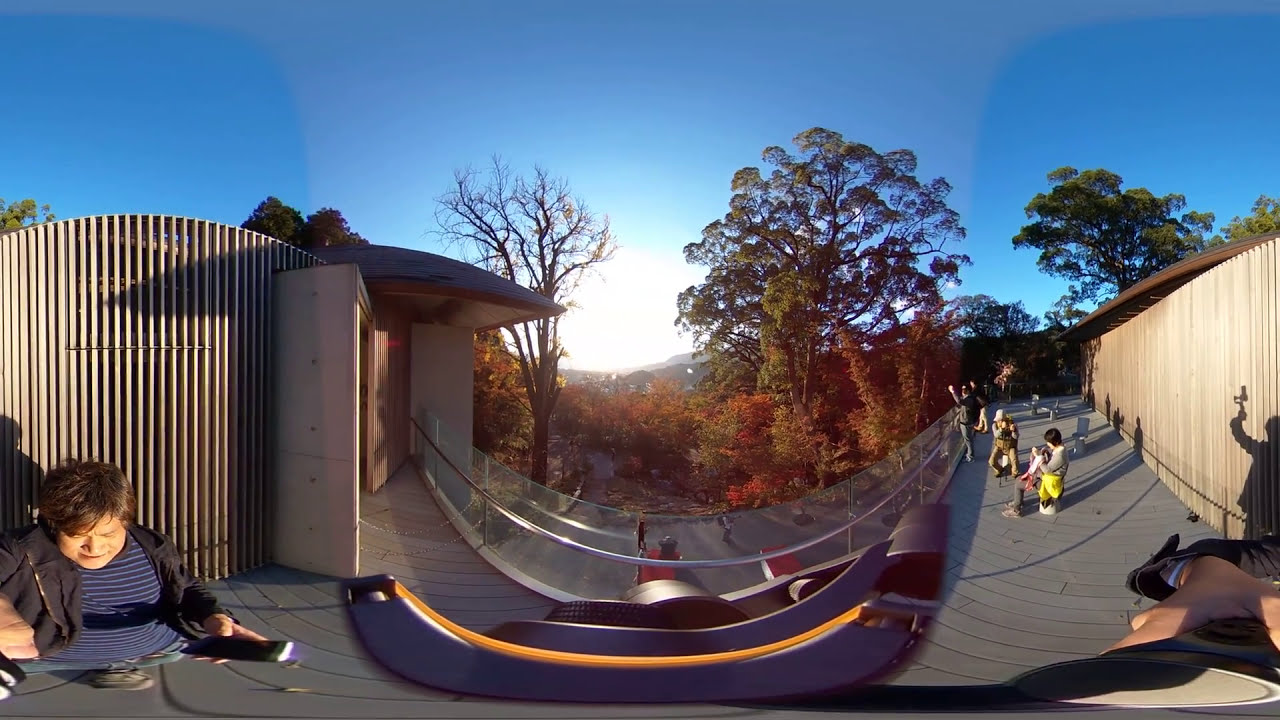This image is a photographic, wide-angle lens shot capturing a bustling outdoor daytime scene at a panoramic lookout deck, where the lens' distortion creates a curved effect. At the forefront, a woman wearing grey pants and a yellow jacket tied around her waist sits in a chair, possibly holding a child. In front of her, a man squats, seemingly taking a photo. Another man stands behind them, looking over a railing towards a sunlit horizon. To the right, you can see the legs of a man in shorts and the shadow of someone holding a phone against the sky. On the left side of the image, a young man in a striped blue and white shirt and a dark jacket holds what appears to be a remote. Nearby, a man stands with a selfie stick. In the distance, the setting sun casts long shadows, silhouetting trees, some still with leaves while one is bare. The scene includes various buildings flanking the deck and a mix of fences and a door, creating a richly detailed, although slightly distorted, view of people enjoying an autumnal vista with trees in hues of red, orange, and green. The background features a wooden fence and rooftops, adding depth to the serene, scenic ambiance.